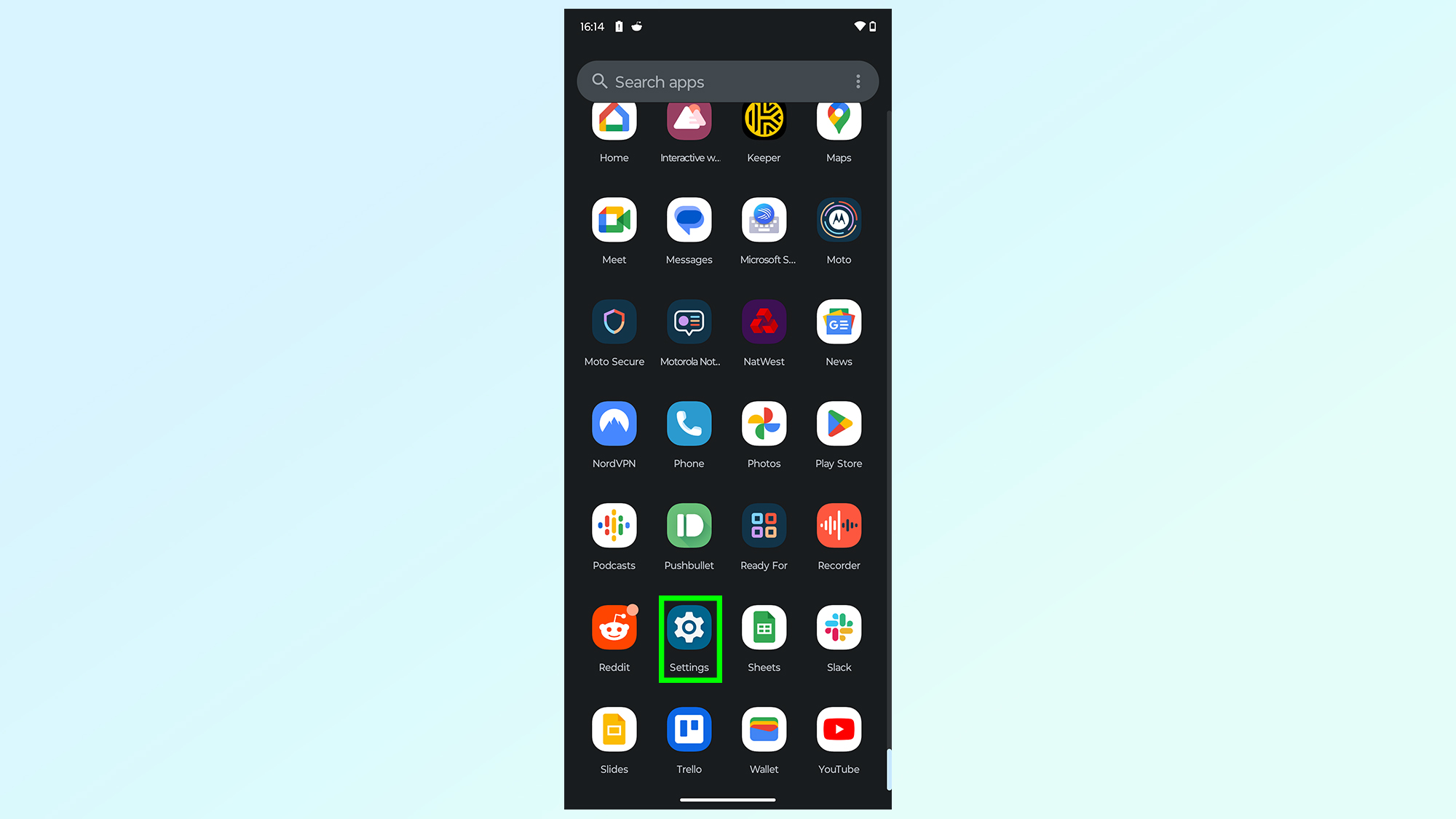In this image, there is a smartphone displaying a portrait-oriented home screen against a light blue background. The smartphone's screen itself has a black background. At the top of the screen, there is a "Search apps" bar.

Various app icons are visible on the home screen, each with distinct colors and designs. Notably, the "Home" and "Cookie Home" apps feature a white icon with red, green, yellow, and blue colors—referred to collectively as "cookie colors." The "Interactive" app icon is maroon and white, while the "Key Pouch" app is designed in black and yellow.

Several other apps also utilize cookie colors: "Maps," "Meet," and "Messages" (which is blue and white). The "Microsoft Swift" app is white and green, and "Motor" is depicted in navy, pink, and purple. "Motor Secure" has a black and red icon, and "Motorola Note" represents a note. The "Netwest" app features purple and red colors, and the "News" app also employs cookie colors.

Further, the "Not VPN" app is blue and white, "Phone" is blue and white, and "Photos," "Play Store," and "Podcast" use cookie colors. The "Pushbullet" app is green and white, while the "Ready For" app is purple, green, red, and orange. The "Ricotta" app is marked in red, white, and black, and the "Ready" app is red and white.

The "Settings" app is gray and white, outlined in a square with green. The "Sheets" app follows a green color scheme, and "Slack" utilizes cookie colors. The "Light" app icon is brown and white, the "Trello" app is blue and white, and the "Wallet" app again uses cookie colors.

Finally, the "YouTube" app is positioned at the bottom left and right, featuring a white and red icon.